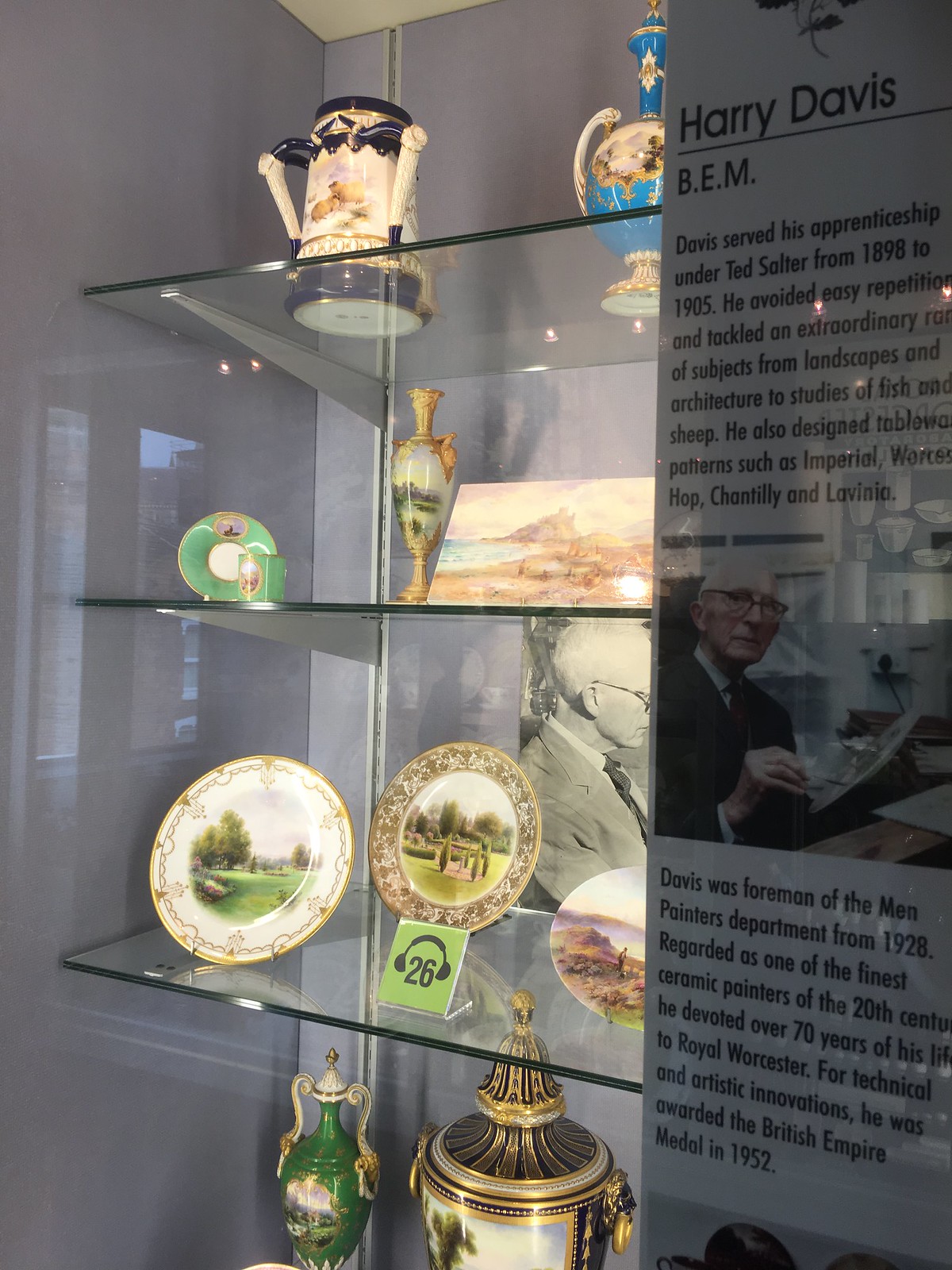The photograph, taken in a museum, shows a highly decorative display of china and pottery on a series of four glass shelves illuminated from within. The top shelf features two intricately decorated vases, while the bottom three are filled with a variety of multicolored antique china, including pitchers, goblets, and plates in hues of white, blue, green, and gold. On the right side of the display, a detailed placard honors Harry Davis, B.E.M. The placard, situated vertically, starts with bold black text reading "Harry Davis" followed by "B.E.M." Below the title are two paragraphs detailing his life and career, notably his apprenticeship under Tan Salter from 1898 to 1905. Between these blocks of text is a photograph of Harry Davis himself, an elderly man with white hair and dark glasses, clad in a black blazer, shirt, and tie, holding a crafted object. This museum exhibit clearly pays tribute to Harry Davis, showcasing his lifetime contributions to decorative arts.